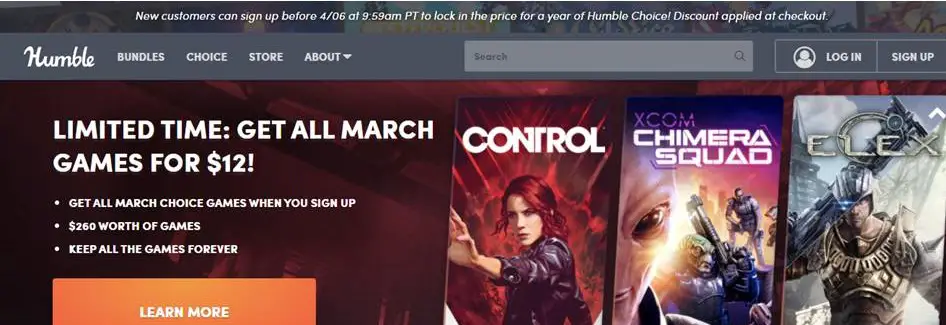This screenshot, captured from the Humble Bundle website on a desktop or laptop, reveals a detailed snapshot of the site's current offerings and interface. At the top, a prominent banner announces that new customers can sign up before April 6th at 9:59 a.m. PT to secure a discounted annual subscription to Humble Choice, with the discount applied at checkout. Below this, the navigation bar features the Humble Bundle logo on the left, followed by menu options including "Bundles," "Choice," "Store," and "About," with a drop-down menu. To the right of these options is a search box, and further right is a "Login/Sign Up" button accompanied by a person icon.

The main content area advertises the Humble Choice subscription plan, a key product promoted by the site. The offer highlights a limited-time deal: new subscribers can get all the March games for $12. This places the screenshot's timeframe in March, though the exact year is unclear. Beneath this offer are three bullet points: "Get all March Choice games when you sign up," "Over $260 worth of games," and "Keep all games forever." An orange "Learn More" button invites further exploration.

Featured prominently are three game titles available through this offer, displayed in rectangular portrait format: "Control," "XCOM: Chimera Squad," and "Elex," each accompanied by their respective logos. This screenshot not only captures the promotional content but also details the layout and navigation elements of the Humble Bundle website.